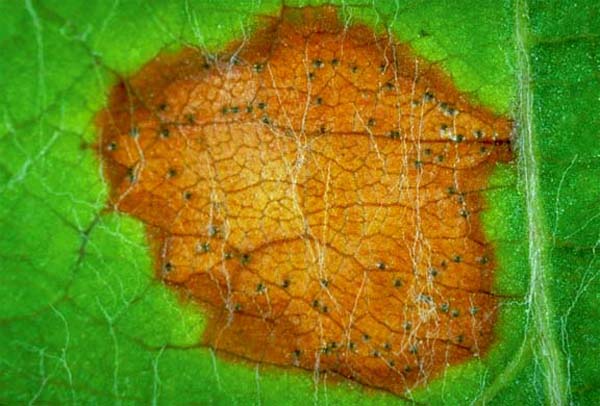This is a full-color, square photograph taken outdoors using natural light. The entire background is filled with the subject itself, which is a green leaf. The leaf showcases a lot of texture and prominent "veins" running through it. The focal point of the image is a large, irregularly shaped brown spot situated dead center, which appears as a dead area of the leaf. Within this brown spot are numerous small black dots that might indicate parasites or some form of decay. Surrounding this brown splotch are additional blackish-green spots. Interestingly, there are also sticky lighter-colored patches and white tendrils extending through the area, suggesting the presence of either disease or another natural phenomenon.